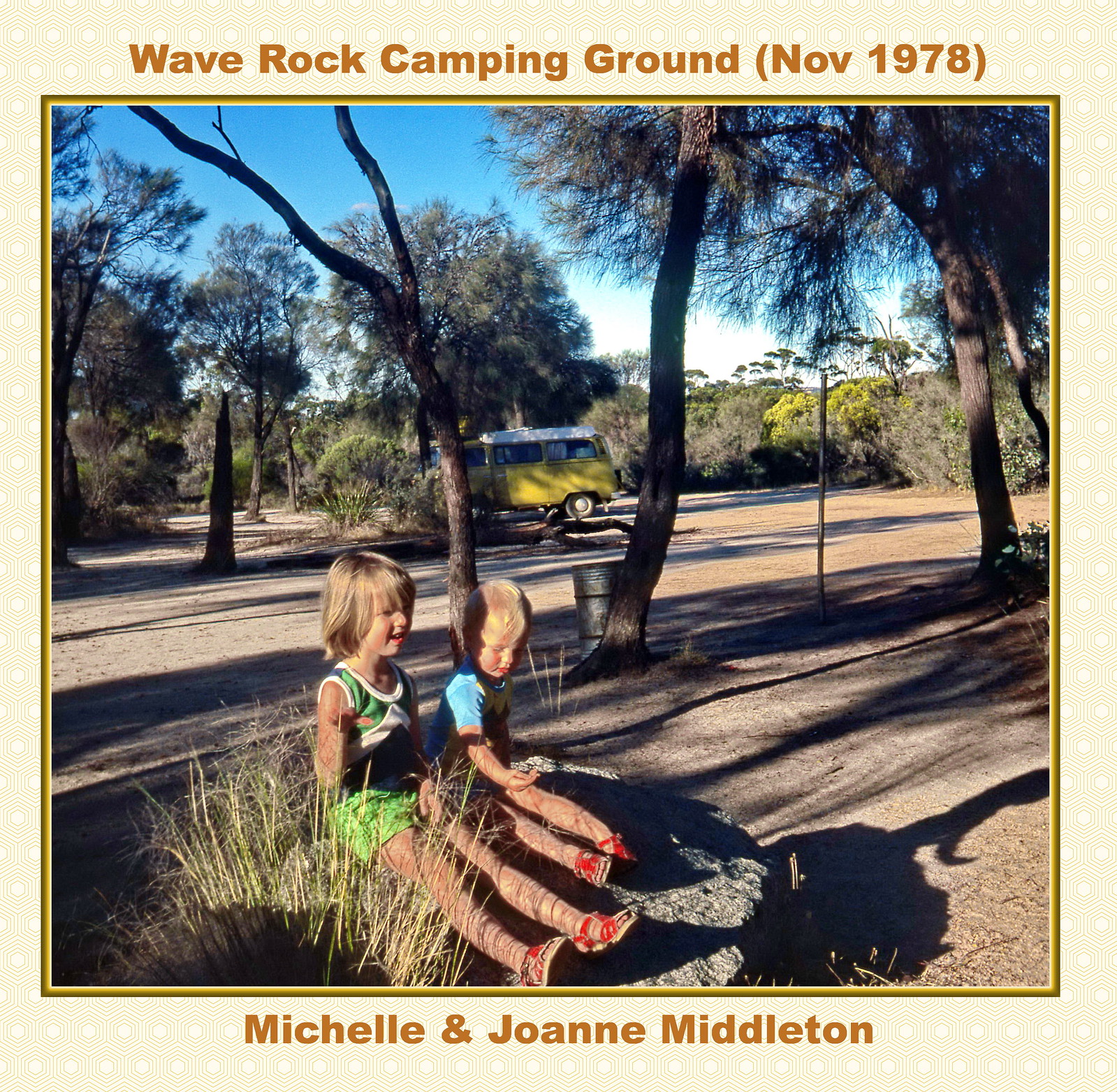This photograph, bordered by a gold trim, captures two young, blonde-haired children, Michelle and Joanna Middleton, sitting on a large, flat gray rock amidst a sunny outdoor scene at Wave Rock Camping Ground in November 1978. The children, appearing to be around two and four years old, are dressed in summer attire, with one in green shorts and a green tank top and the other in a blue t-shirt, both wearing red sandals. The late afternoon sunlight casts their shadows on the rock, and tall green and tan grasses grow nearby. Surrounding them is a landscape of well-kept dirt pathways and fully-leafed trees, showcasing their green foliage against the vivid blue sky. In the far background, a white-topped, yellow and greenish VW camper bus is parked, adding a nostalgic touch to the picturesque setting.